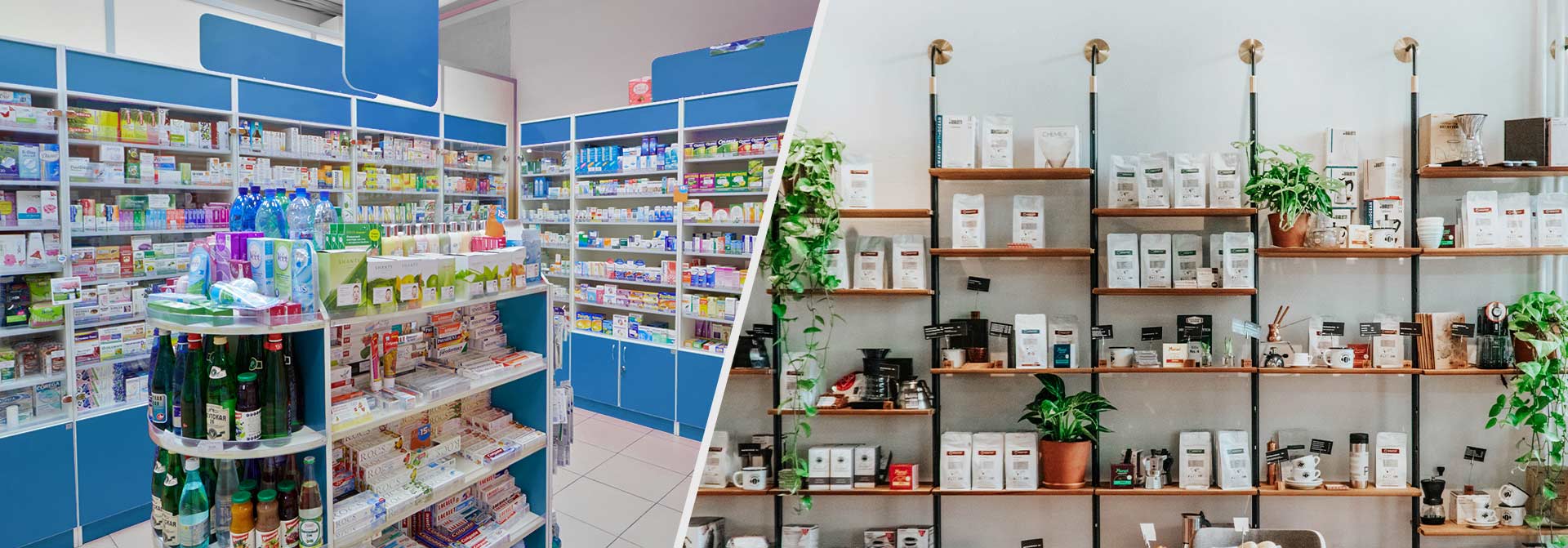The image features contrasting side-by-side depictions of two distinct storefronts. The left side showcases a traditional pharmacy, characterized by its antiseptic blue and white color scheme. It features blue painted walls and shelves neatly lined with bottles and packets of medicine. A white floor and other white elements around the shelving units enhance its clinical, commercial atmosphere. In the center aisle, there's a small stand displaying products. The modern right-hand side presents a boutique-style shelf setup, exuding a homely and intimate feel. It features brown shelves adorably decorated with potted plants, neatly sorted items, and some gold accents. Both sides have white walls, but the right side is adorned with aesthetically placed products, evoking a cozy, salon-like ambiance.